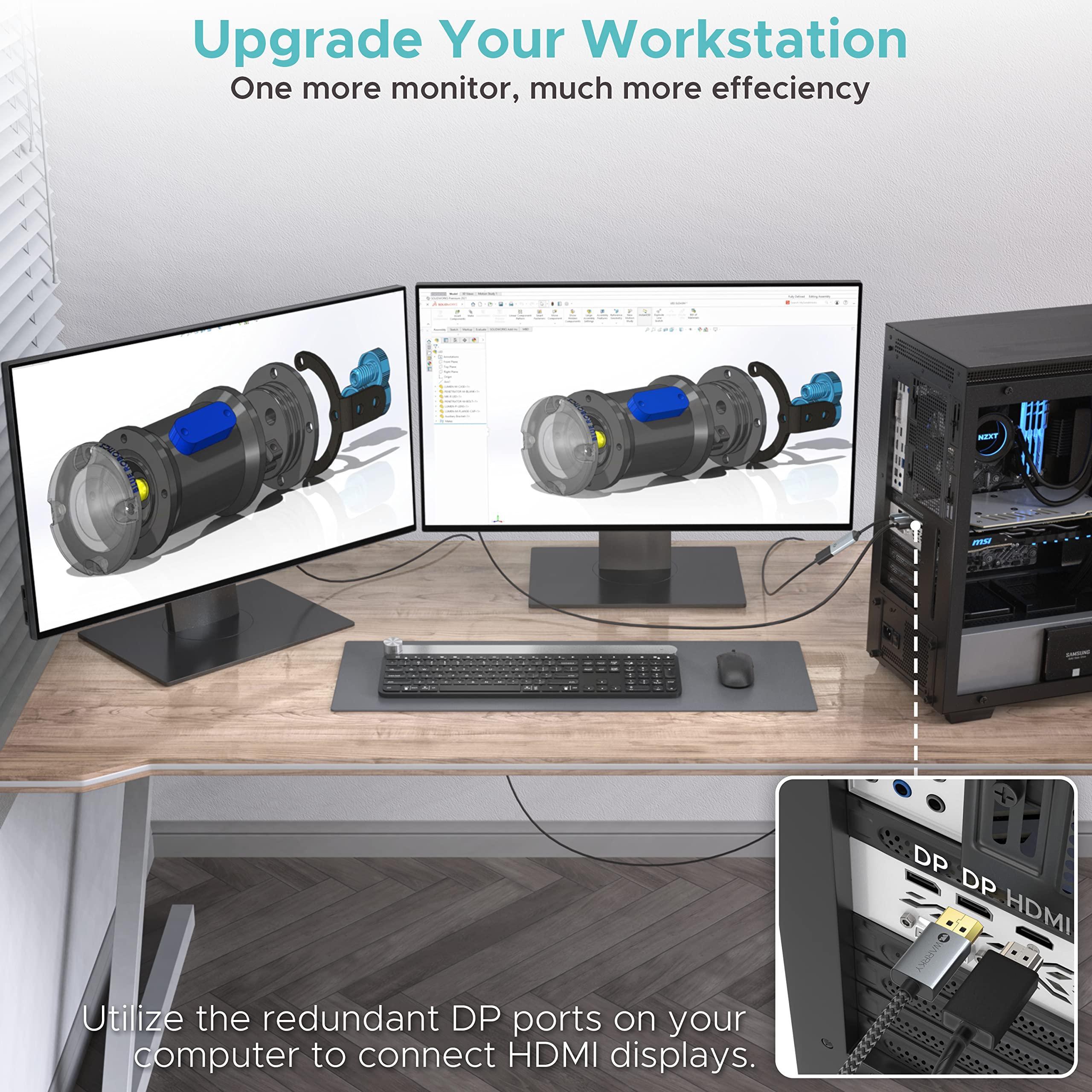The image is a professional photograph of a neatly organized office workspace, likely used for an advertisement or promotional poster. It captures the corner of a room with pristine white walls and sleek, light gray wooden floor tiles. The centerpiece is a nice wooden desk outfitted with two equally sized computer monitors. The setup includes a black keyboard and a mouse arranged on the desk, which sits before a powerful desktop unit equipped with advanced liquid cooling and a high-end graphics card. 

The workspace is illuminated softly, highlighting the clean and modern aesthetic. To the left, there's a window with vertically drawn white blinds, adding a touch of natural light. The text on the poster begins at the top in prominent gray letters with the message, "Upgrade your workstation." Beneath it, in black text, it states, "One more monitor, much more efficiency." This emphasizes the productivity benefits of having an additional monitor, suggesting that once you experience it, you'll find it hard to revert to a single screen setup.

At the bottom, in white text against a background, the poster reads, "Utilize redundant DP ports on your computer to connect HDMI displays," advocating for optimal use of available ports. Adjacent to this text, there’s a detailed diagram showing a close-up view of various cables and where they should be connected on the desktop unit, which includes HDMI and DP ports. The monitors display an exploded view of a technical device, possibly a camera, showcasing its internal components and design schematics, reinforcing the high-tech and efficient theme of the advertisement.